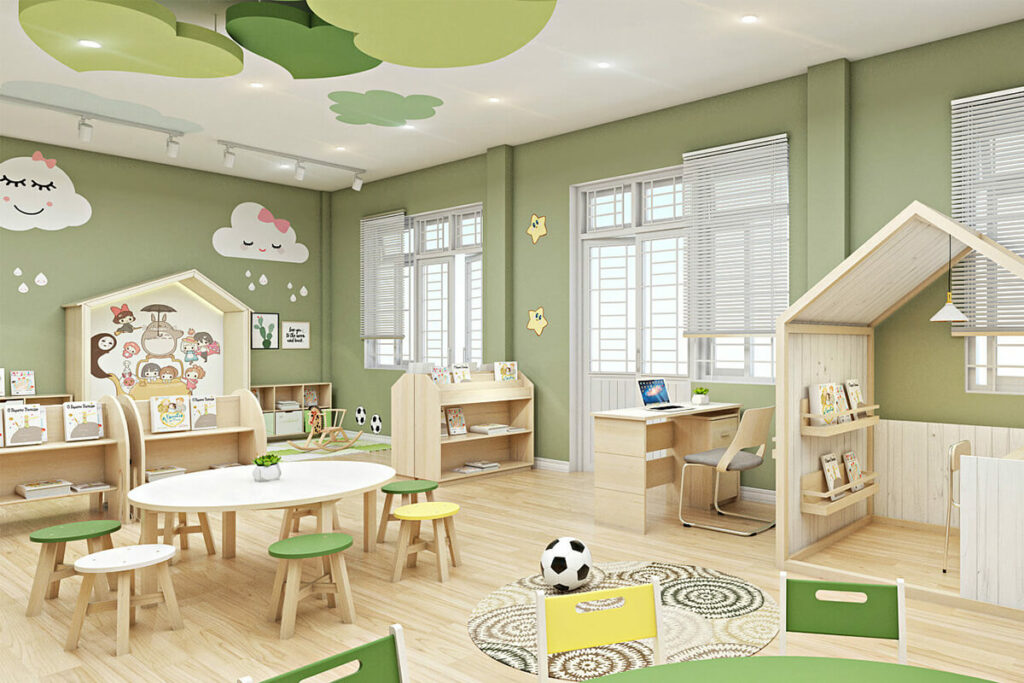The image depicts a charming and meticulously designed daycare center or preschool with an inviting atmosphere. The interior is characterized by matcha green walls and light, airy wood flooring. Most of the furniture and structures within the space, including tables, chairs, and bookcases, are crafted from the same light-colored wood, contributing to a cohesive and harmonious aesthetic.

The décor features playful elements such as cartoon-like clouds with faces painted on the walls and three heart-shaped ornaments suspended from the ceiling, also in matcha green. In one nook, chibi-style characters from Studio Ghibli films, including Totoro, the witch girl from Kiki’s Delivery Service, and creatures from Spirited Away, add a whimsical touch. The color palette includes soothing greens, mellow yellows, and crisp whites.

The center is well-equipped with several play areas and child-sized bookcases brimming with children’s books. There’s a cozy playhouse where children can retreat to read under a small lamp, fostering a quiet and serene environment for relaxation. Additionally, a desk with a laptop suggests opportunities for interactive learning games. A soccer ball on a mat indicates space for physical play. The well-coordinated design and carefully thought-out details make this daycare center both functional and aesthetically pleasing.